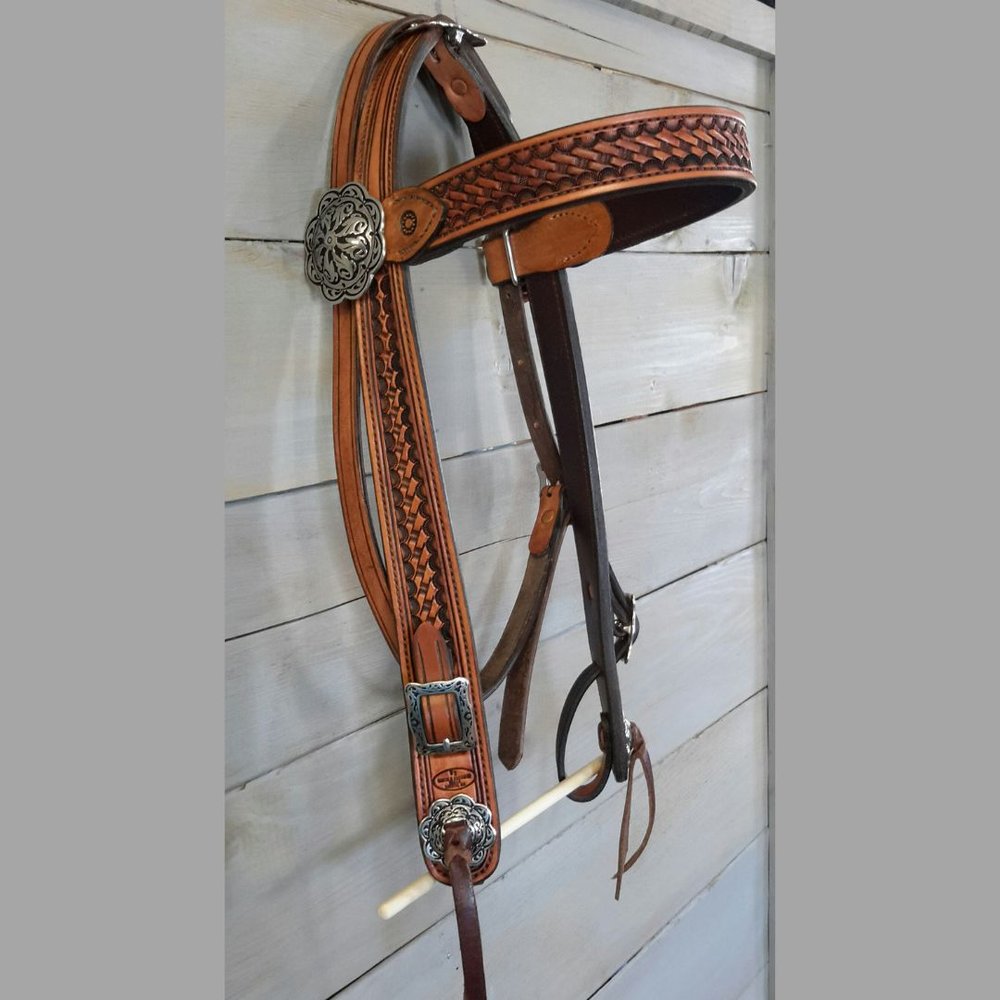The image features a detailed close-up view of a brown leather harness designed for equestrian use, placed on diagonally arranged white wooden planks, possibly part of a table or flooring. The harness includes multiple straps, with two prominent ones forming an upside-down U-shape, adorned with various grommets and decorations. There are silver grommets on the corners where the straps loop over, a brass grommet at the front, and another silver grommet at the end, as well as some decorative metal flower-like elements. A wooden dowel stretches across the bottom of the harness, possibly to mimic how it would sit around a horse's mouth or under its neck. The harness is hung neatly, suggesting it is either displayed or stored for future use. The lighting in the image comes from the right, casting subtle shadows that emphasize the textures and materials of the harness and the wooden surface beneath it.